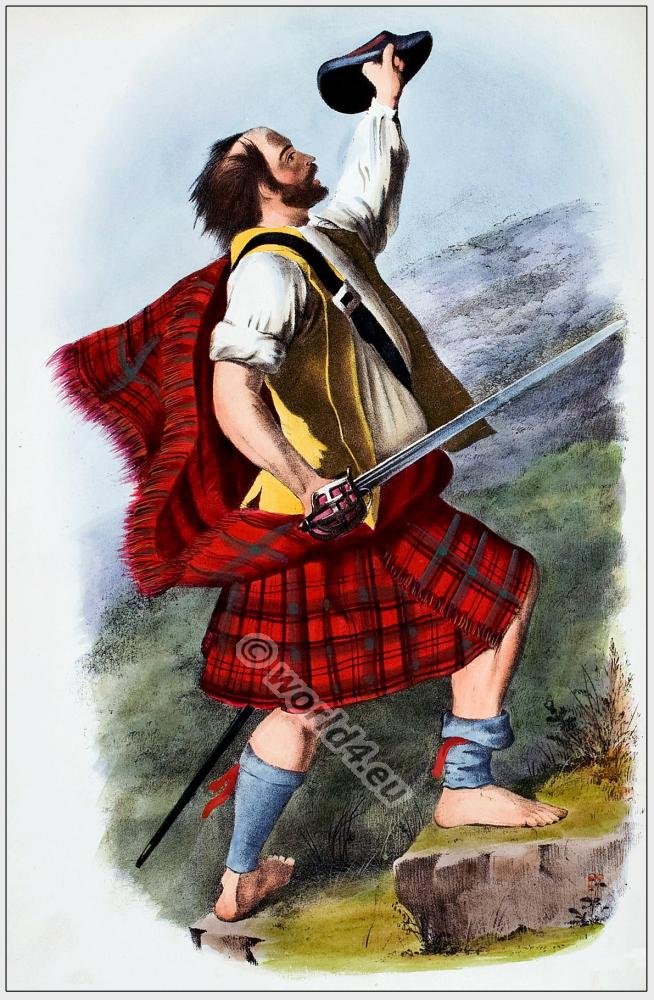The image is a detailed cartoon illustration of a presumably Scottish man, identifiable by his traditional attire. He is light-skinned with noticeable male pattern baldness, complemented by long black hair at the back of his head and a full beard. The man dons a red plaid kilt with green and black lines, and a white long-sleeve cotton shirt with the sleeve on his right arm rolled up to his bicep. Over the shirt, he wears a yellow vest and a black leather strap with a silver buckle across his chest, possibly connected to a bag or sword sheath that is partially visible near his left foot. His feet are bare, but he is adorned with blue leg warmers, though the one on his right leg has slipped down to his ankle.

In his left hand, he holds a blue beret, raised in the air as if waving, and in his right hand, he brandishes a sword. His stance suggests he is in mid-motion, possibly climbing a rock formation resembling steps, or positioned on the side of a mountain. The background hints at an outdoor setting with grass or moss-covered terrain. His animated pose and detailed attire paint a vivid picture of a spirited Scotsman in a moment of action.